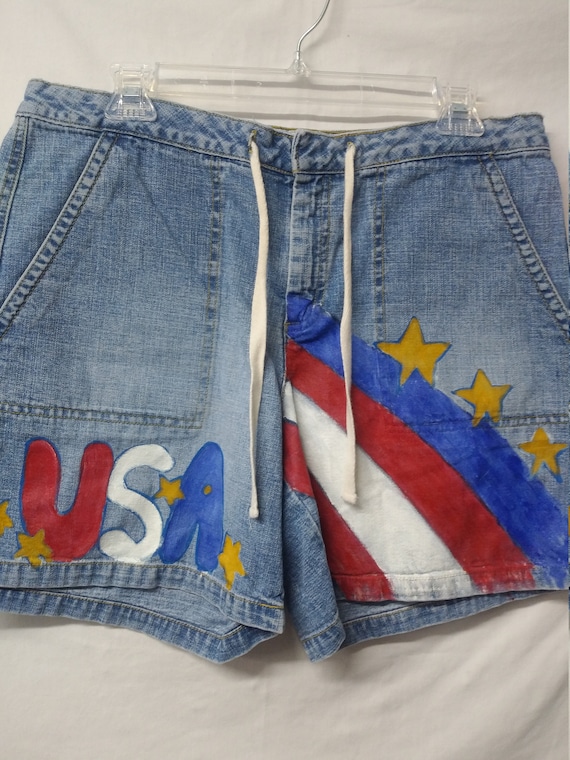In this image, a pair of women's jean shorts is prominently displayed on a slightly wrinkled white sheet, creating a neutral backdrop. The shorts are neatly hung on a clear plastic hanger with metal hook, secured by clips on each side. The denim is white, featuring distinct design elements. On the left leg near the seam, "USA" is boldly emblazoned in patriotic tones—red for the "U," white for the "S," and blue for the "A"—accompanied by several gold stars. To the right side, there's a striking pattern resembling a flag, with blue at the top, followed by red, white, and ending with red closest to the crotch. This section also has three golden stars that marginally overlap with the blue stripe. Finishing the look, white drawstrings hang from each side of the waistband, adding a casual, functional detail to the stylish shorts.